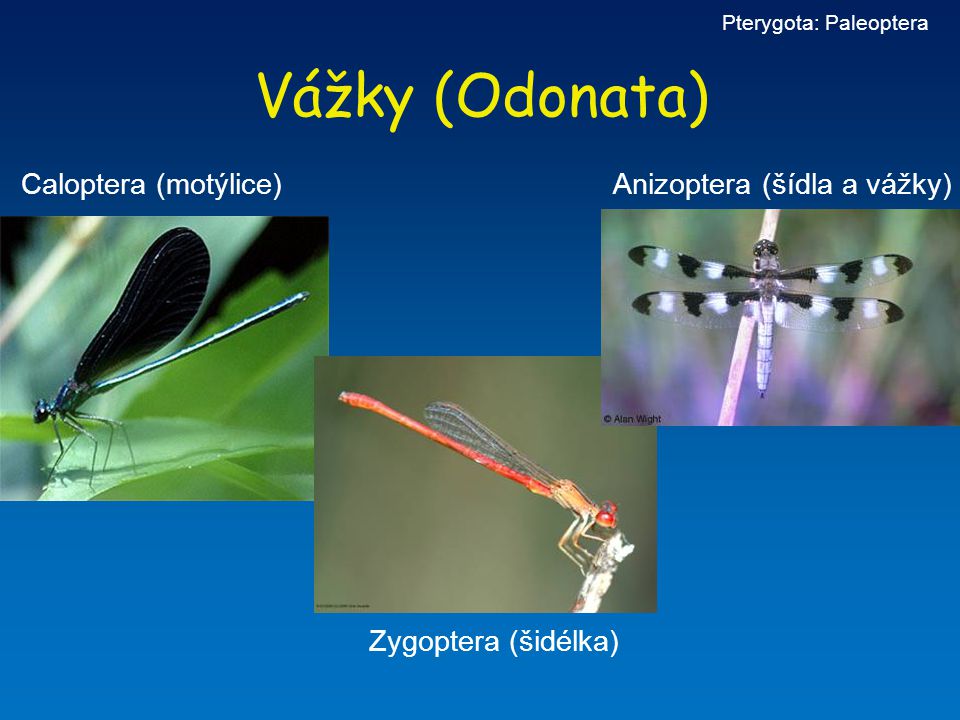The image features a digital composition that resembles a PowerPoint slide with a blue background, which transitions from a darker navy blue at the top to a lighter blue at the bottom. In the top right corner, the white text "PTERYGOTA: PALAEO-PTERA" is prominently displayed. The central title in yellow, styled in Times New Roman font, reads "VAZKY (ODONATA)." This slide showcases three distinct images of dragonfly-like insects, each accompanied by a unique label in a foreign language.

On the left, the first image depicts a dragonfly with black wings and a silvery, glistening abdomen, perched on a green leaf. The label above this image is "CALOPTERA (MUTILISE)." The middle image features a dragonfly with an orange body, red eyes, and clear wings, settled on a twig or branch; its caption reads "ZIGAOTURA (CEDELCA)." The rightmost image shows a dragonfly with striking black and white striped wings, a white abdomen, and a black head, also perched on a twig. This insect is labeled "ANISOPTERA."

The blue background, varying in shade, the detailed insect images, and the captions indicate this might be an educational slide or informational graphic related to entomology, displayed in a language that seems difficult to read but adds a scientific context.